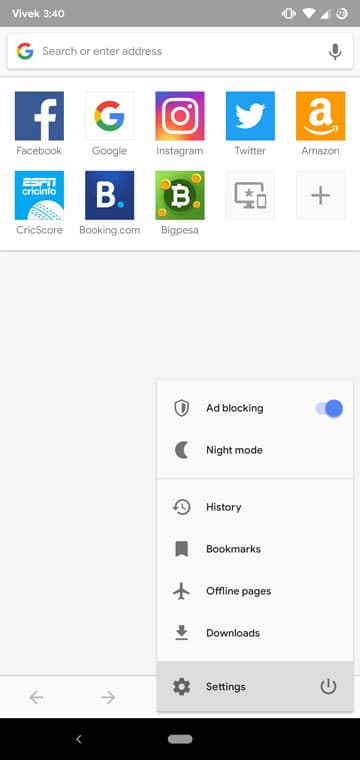This is a detailed screenshot from a mobile phone interface. At the very top, a gray notification bar displays the text "Vivec 340" on the upper left. On the right end of this bar, several icons are visible: a vibration icon indicating vibration mode is on, a full mobile signal icon, and a Wi-Fi icon showing a strong connection with almost all bars filled except one.

Below the notification bar, a white rectangular search field is present. On the far left of this field is the Google 'G' logo. Within the field, gray text reads "Search or enter address," and on the far right, a gray microphone icon is visible. 

Beneath the search field, several commonly used app icons are displayed in a horizontal row. These include the Facebook, Google, Instagram, Twitter, Amazon, ESPN Cricinfo, Booking.com, and BigPesa icons. There is also a small plus sign at the end of the row, indicating the option to add more icons.

Further down, a menu is open against a white background. At the top of the menu, "Ad Blocking" is displayed, accompanied by a shield icon, indicating that ad blocking is turned on. Below this, "Night Mode" is listed with a moon icon. The next item is "History," indicated by a clock icon, followed by "Bookmarks."